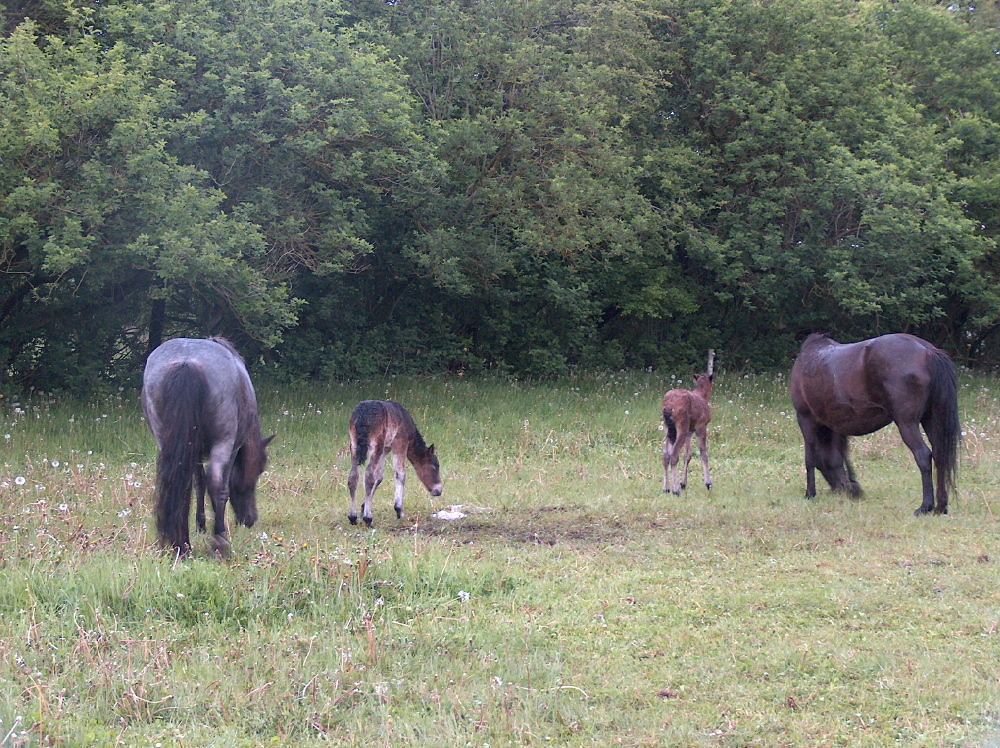A vibrant photograph captures a serene scene of four animals grazing in a grassy field, surrounded by lush, green trees. In the foreground, two full-grown horses with dark bodies and long black tails stand majestically. One of these adult horses has darker fur, while the other has a brownish-black coat. Each stands near a smaller companion, possibly ponies, grazing beside them. One pony displays a multicolored coat of black, brown, and white, particularly visible on its legs, while the other pony is predominantly brown with a sleek black tail. The grass beneath their feet is a mix of lush green interspersed with patches of brown and dirt, dotted with dandelions and various other small plants. The photograph offers a rear view of the animals, with three of them focused on their grazing, heads bent down, while the pony on the right gazes directly ahead. The setting is illuminated by daylight, adding to the overall tranquility and natural beauty of the scene.